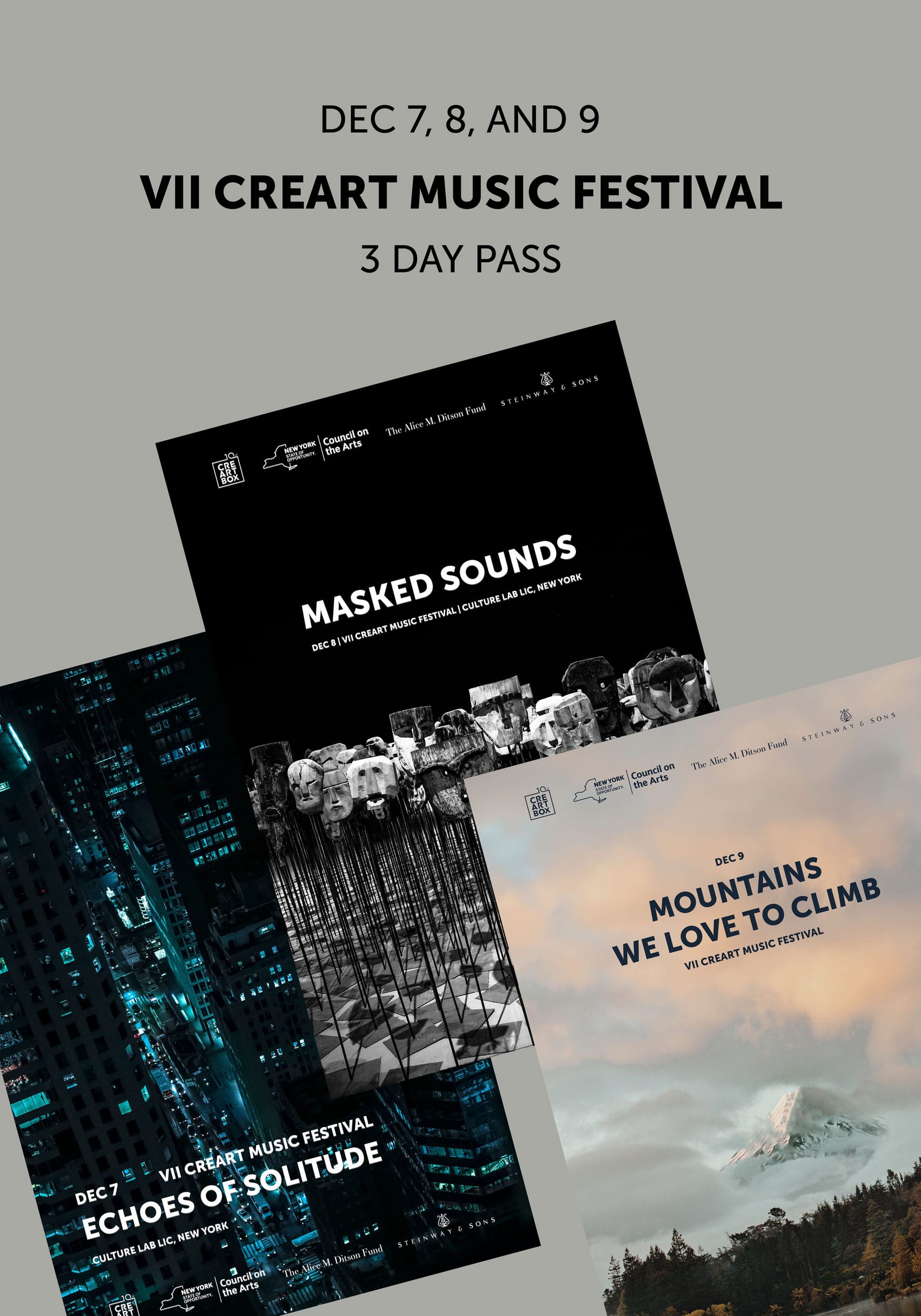This detailed print advertisement promotes the VII Create Music Festival, which spans December 7th, 8th, and 9th. The main backdrop is gray with black text announcing a "Three-Day Pass" for the festival. Below this heading, there are three smaller sub-advertisements, each detailing one of the festival's themed nights.

The first sub-advertisement, set against a cityscape background, promotes "Echoes of Solitude" on December 7th at Culture Lab LIC, New York. The second sub-advertisement, featuring a black background with eerie masks on sticks, highlights "Masked Sounds" taking place on December 8th, also at the Culture Lab LIC. The final sub-advertisement, depicting majestic mountains over a forest, announces "Mountains We Love to Climb" taking place on December 9th. Each sub-advertisement distinctly conveys the unique visual and thematic elements of their respective events within the festival.